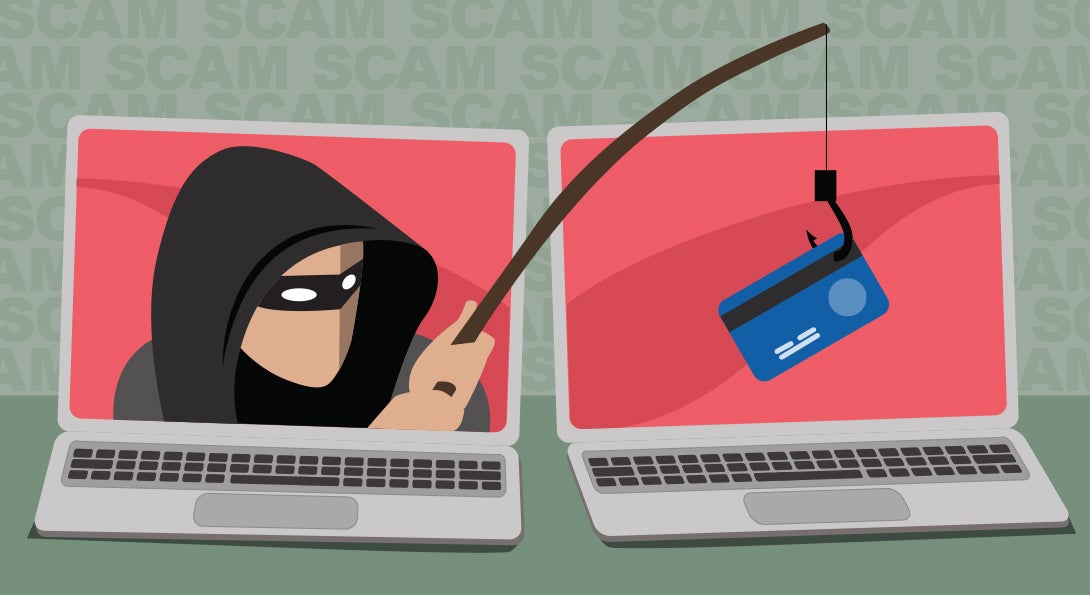The digital artwork features a striking gray background repetitively inscribed with the word "scam" in dark gray letters. At the forefront, two nearly identical laptops are positioned side-by-side on what is likely a representation of a green table. Both laptops display red screens. Emerging from the screen of the left laptop is a Robin Hood-esque figure clad in a black hood and a black mask with featureless white eyes, lacking any visible nose or mouth. This simplified figure, characterized by solid colors, holds a brown phishing line in both solid-colored hands. The line descends into a big black hook that suspends a blue credit card, which is being extracted from the right laptop. The keyboards of the laptops are also designed with solid colors against the contrasting gray background of each bottom section. The overall theme vividly depicts the act of phishing, with the left screen's masked figure illicitly retrieving a credit card from the adjacent laptop.